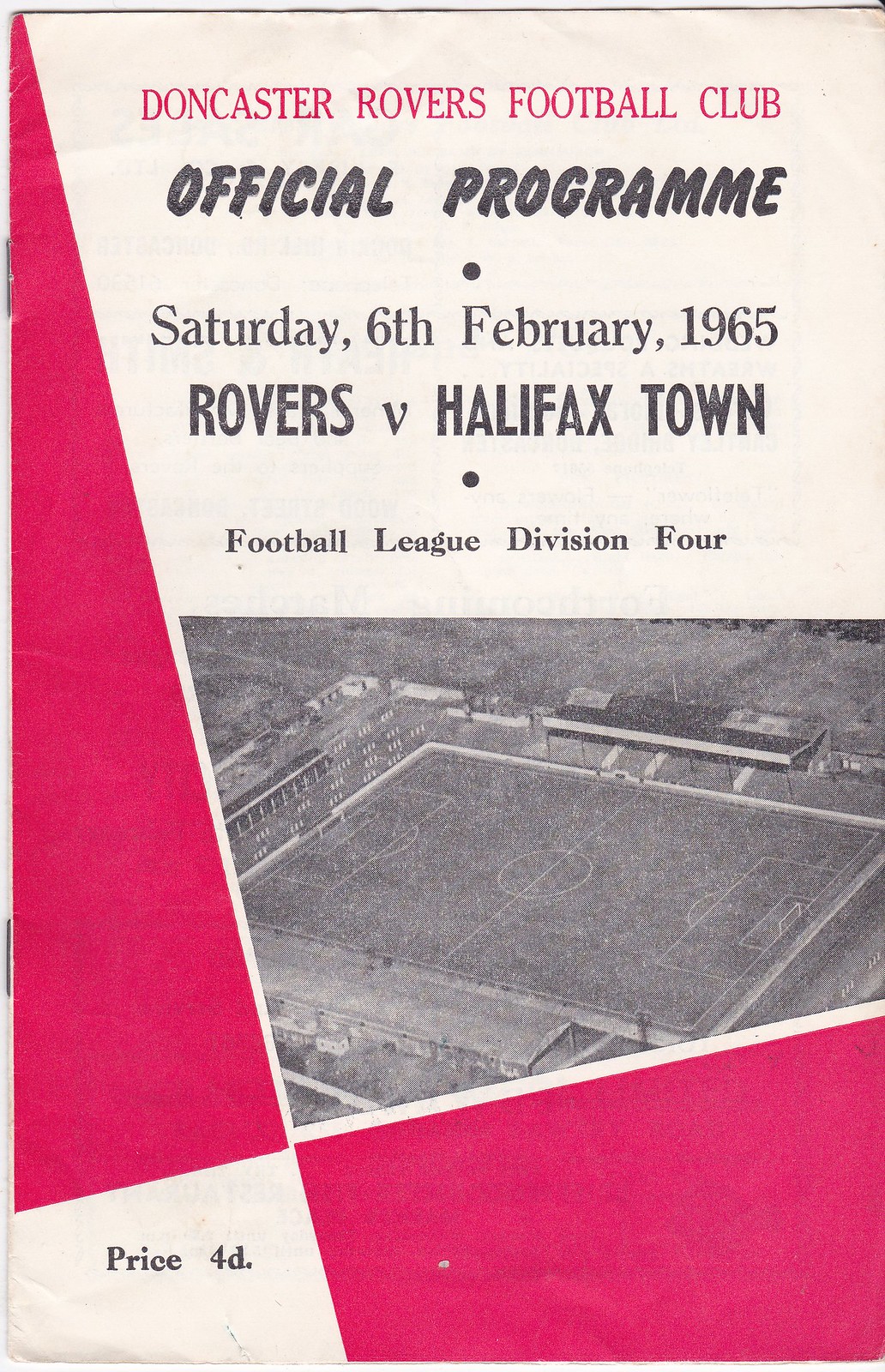The cover of the old-timey Doncaster Rovers Football Club program from Saturday, 6 February 1965, features bold red capital letters spelling out "Doncaster Rovers Football Club" atop a white background. Directly below, in black capital letters, it reads "Official Program." Following that, in smaller black letters, the date "Saturday, February 6, 1965" is noted. Continuing downward, it states "Rovers versus Halifax Town" and "Football League Division 4" also in black capital letters. The left side and the bottom right portion of the cover are framed by a red background, giving it a checkered appearance. In the bottom left corner, there is a small white area with "Price 4D" written in black. Centrally placed on the page is a faded, black-and-white aerial image of a football field, complete with visible stands and field markings, providing a nostalgic glimpse into the historical sporting event.